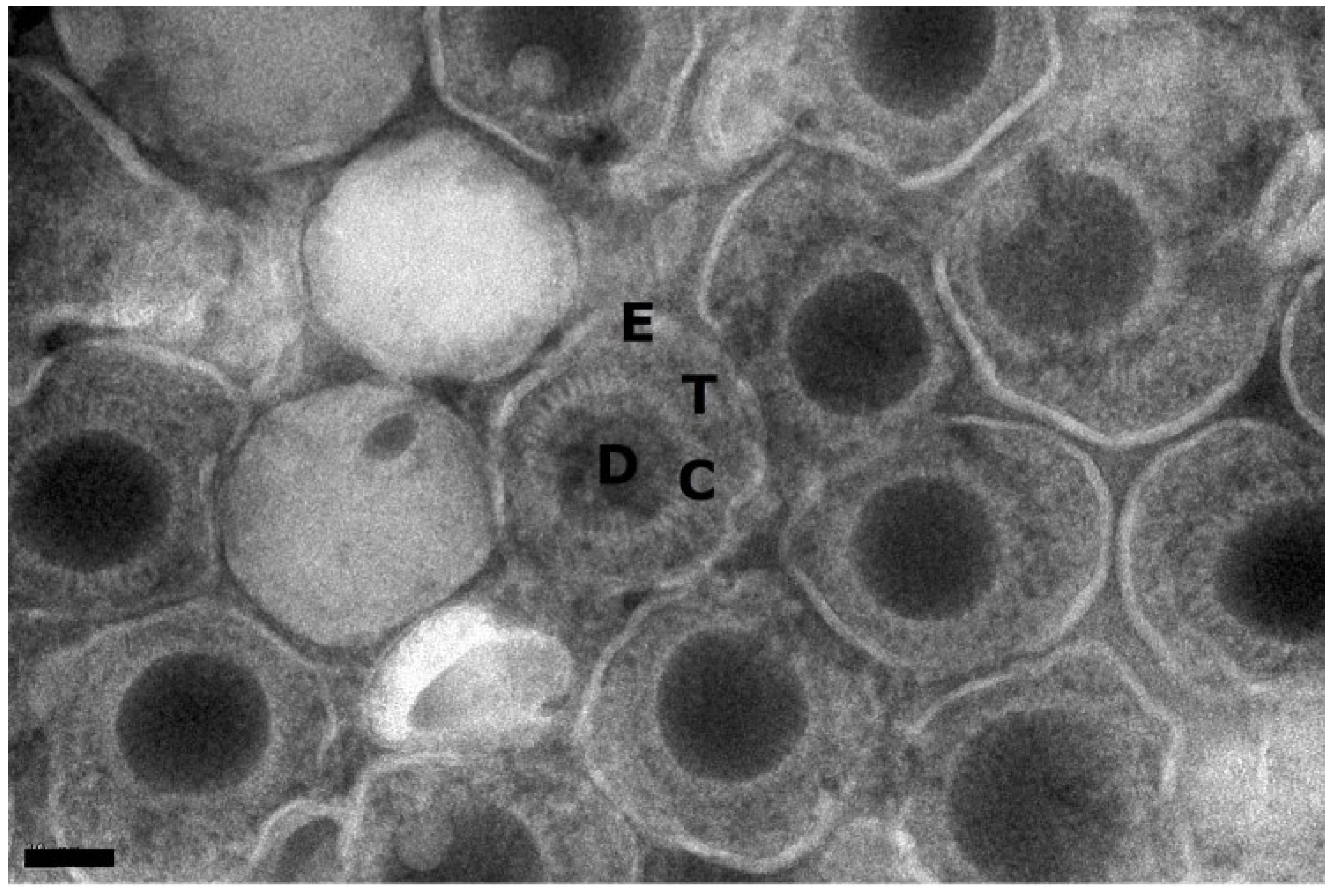The image is a high-resolution, black-and-white photograph taken through a microscope, likely an electron microscope, depicting numerous round animal cells. In each cell, the cell membrane and nucleus are clearly visible. Distinctively, in the center of the image, there are four superimposed letters: E, T, C, and D. The exact significance of these letters is unclear, but they appear to mark or denote specific features or an event within the photo. Additionally, there is a singular, solid white cell near the upper left quadrant. The surrounding background consists mainly of dark black circles, suggesting cellular structures possibly stained for clarity. The absence of a detailed caption leaves the precise context and scientific purpose of the image open to interpretation.